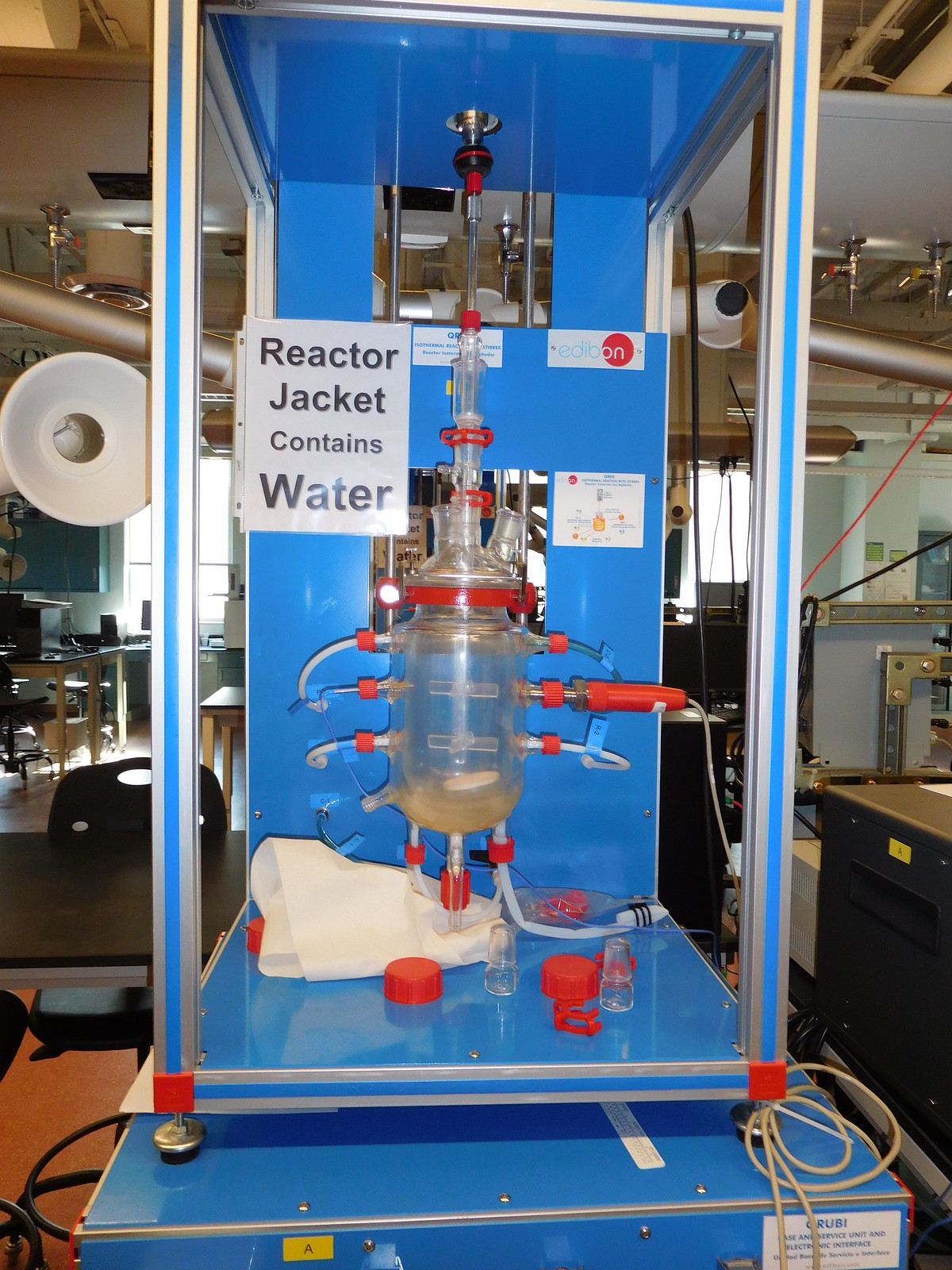The image features a piece of scientific equipment labeled "Reactor Jacket - Contains Water," prominently situated at the center of the scene. The apparatus consists of a large glass container with a canister connected by a red rubber band, various small glass tubes, and three hoses extending from the sides. The setup is partially encased in plexiglass on the front and sides, with a blue metal frame and additional metal pipes at the back. The machine rests on a small metal platform in what appears to be a laboratory environment. Scattered red caps are visible on the platform, and to the left of the apparatus is a strobe light. The background reveals lab desks and other laboratory equipment amidst various scientific gear. The image is devoid of any individuals or identifying information such as a date or location, and the scene seems to be captured indoors, possibly in a science classroom. Dominant colors in the image include blue, white, yellow, red, gray, black, brown, and silver.